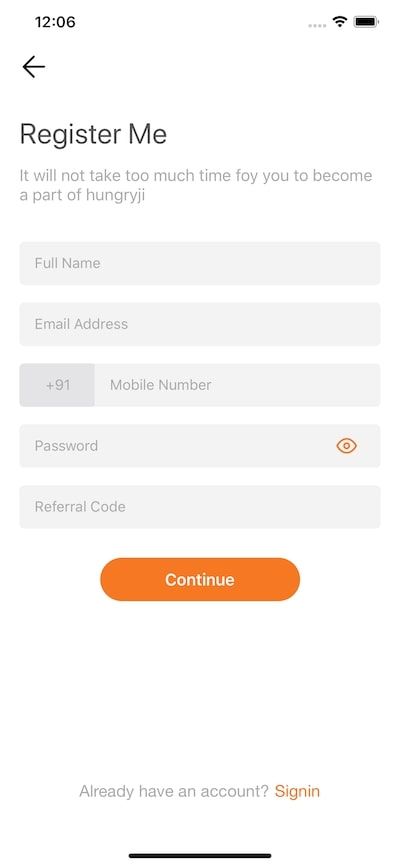The image displays a mobile device screen showcasing an application or website interface. At the very top left of the screen, there's a timestamp reading "12:06" in black font. To the right of the timestamp, four dots indicate the data signal, suggesting the device's service might be turned off or there is no service. Further right, there's a black Wi-Fi symbol, and next to it, a black battery icon indicating about 90% charge.

Beneath this status bar, on the left side, an arrow points left, indicating the option to return to the previous page. Below the arrow, the header "Register Me" is prominently displayed in black text. Subtly beneath this, in smaller gray text, it reads, "It will not take too much time for you to become a part of HungryJI."

The main part of the screen features a registration form. The form includes fields to fill in the full name, email address, and mobile number. The mobile number field is prefixed with a darker gray rectangle displaying "+91" in its center. There's also a password field, with an orange outline of an eye icon to its right. Below these fields, there's a spot for a referral code.

Towards the bottom center of the screen, a bold, oval-shaped button with an orange background and white text states "Continue." At the very bottom, in light gray text, it asks, "Already have an account?" To the right of this question, an orange clickable link reads "Sign In." A short, centered black line separates these sections, adding a finishing touch to the layout's organization.